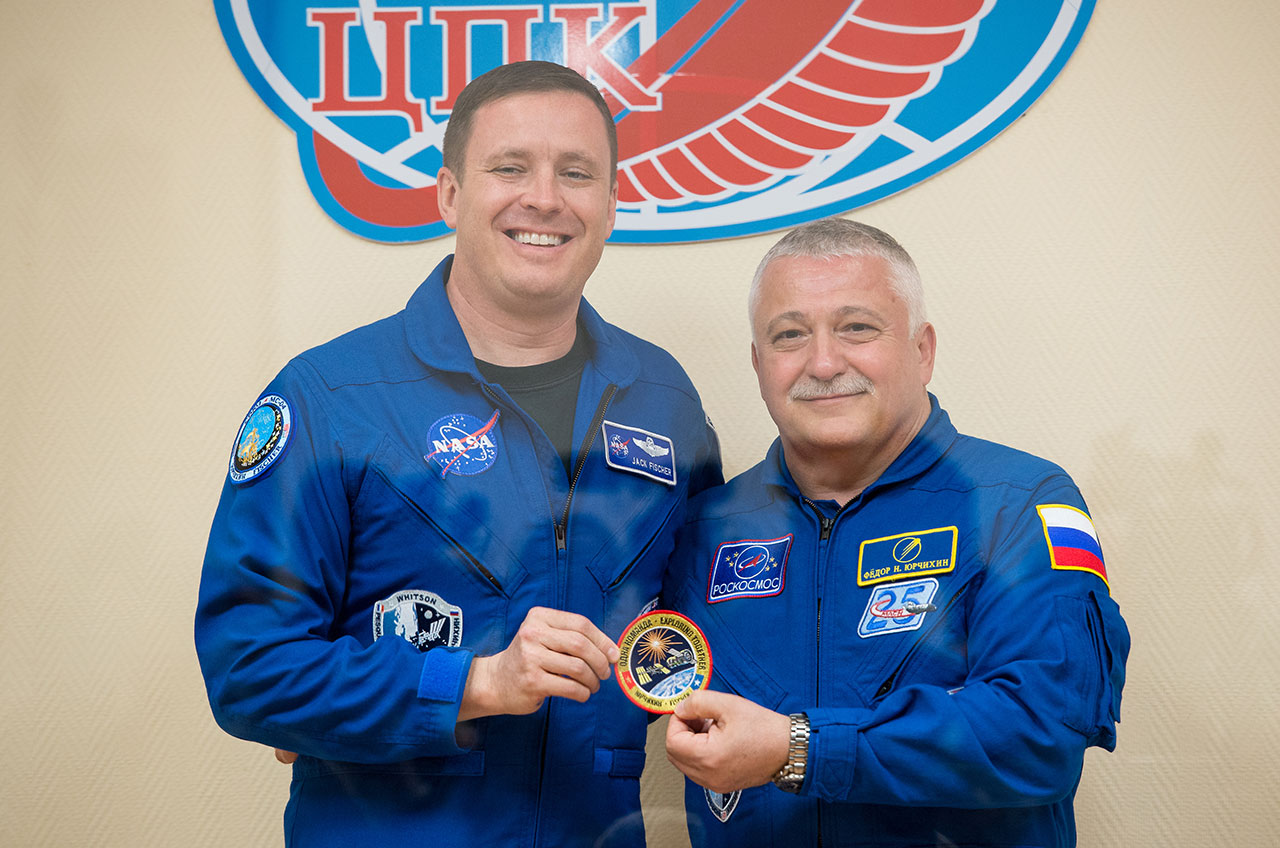In this photograph, two astronauts stand side by side against a backdrop featuring the Russian term "UNK" in red and blue. Both men are clad in blue flight suits adorned with multiple patches indicating their affiliations. The taller astronaut to the left, identified as Jack Fisher from NASA, is in his late 20s or early 30s, with short brown hair and an open smile. His suit prominently displays a NASA patch. The shorter astronaut to the right is likely a Russian cosmonaut, identifiable by the flag patch on his left shoulder, featuring stripes of white, blue, and red with a yellow border. He appears to be older, possibly in his mid-50s, with gray salt-and-pepper hair and a stockier build. He sports a closed-lip smile and wears a watch on his wrist. Both men are holding a patch together, signifying some sort of international cooperation or fellowship, possibly linked to a joint space mission. They are both grinning, radiating a sense of camaraderie and mutual respect.